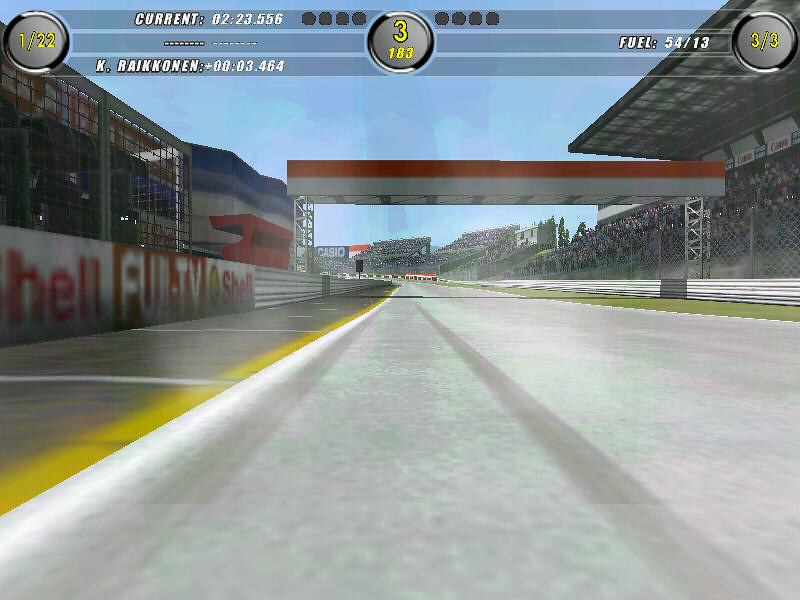This detailed image from a racing video game portrays a Formula 1 track viewed from a first-person perspective. The gray road stretches deeply into the image, beginning from the left corner and veering slightly left halfway up and out of view. The right-hand side of the track features a white and red striped border adjacent to a small concrete parking area. Midway up on the left side, a side guardrail is visible, alongside a white square advertisement with red lettering reading "Hell," followed by another advertisement. Further up, there is a gray cage on the left side. The right side of the road showcases green grass, a barrier, and then a fence enclosing a digital crowd in the far background.

The track includes a prominent overpass with a red and white structure extending across the road, typically where the flagger stands. Next to the right-hand side, there is an awning for spectators to sit under. The background reveals stands filled with more digital crowds, underscored by a blue sky. Advertisements of "Shell" and "Fuji TV" along with other branding points towards Formula 1 racing. Additionally, there is a noticeable advertisement for Casio in a building across the racetrack. Overhead information displays the player’s current position, remaining fuel, and racing times. The finish line is prominently visible, reinforcing the competitive racing atmosphere of this immersive game.